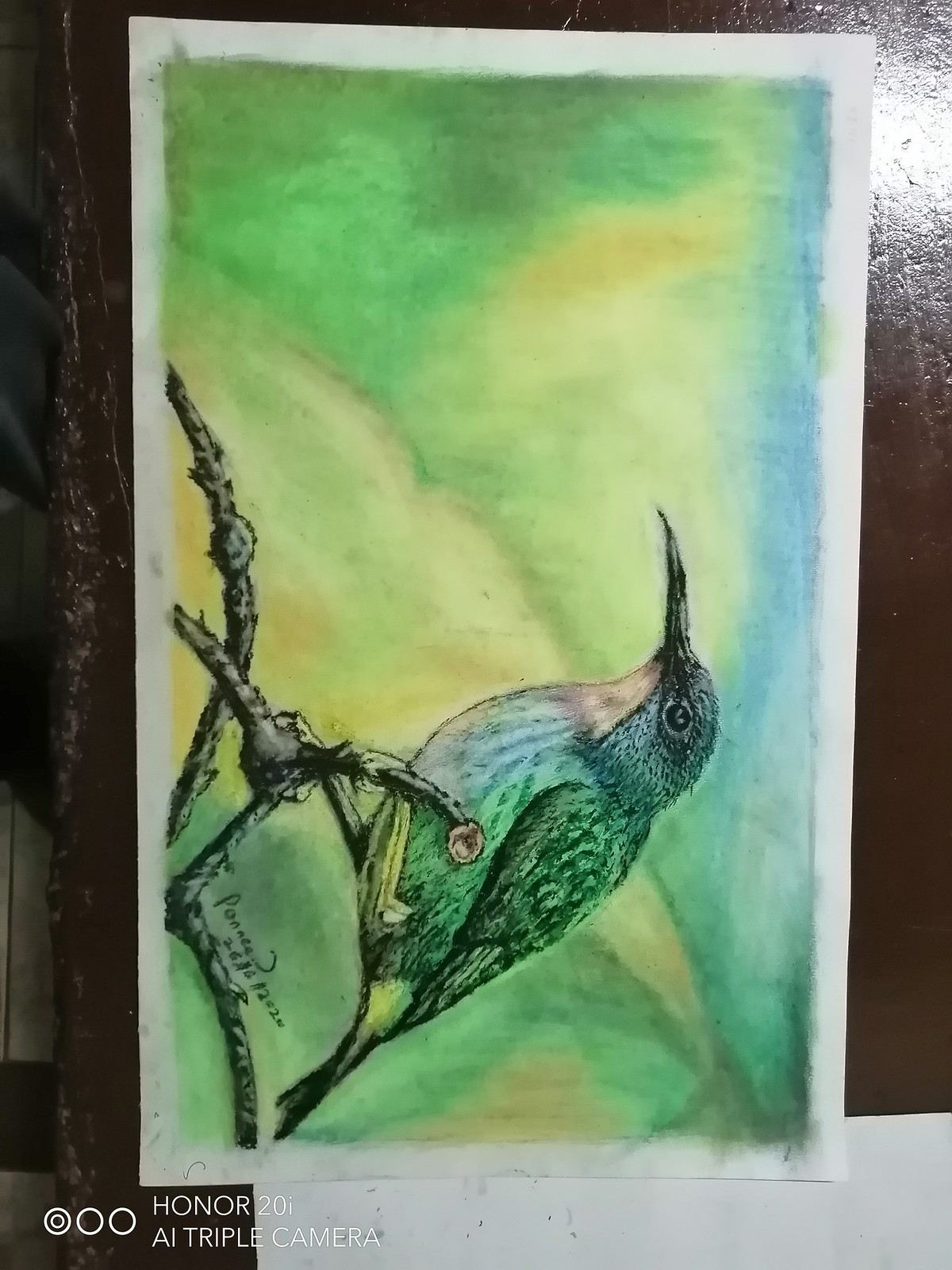This photograph showcases a meticulously hand-created watercolor painting of a hummingbird, artistically rendered on white paper and resting on a brown table. The painting captures the hummingbird perched calmly on a set of twigs, detailed with fine black ink. The bird features a vibrant mix of green, pale yellow, and black, highlighted with subtle purple and blue hues on its wings and belly. It has a long beak, similar to that of a hummingbird, and a white breast with a lightly-colored beige throat and striped chest. The bird's eye is visible, adding a sense of tranquility to its posture. The background blends soothing shades of blue sky with greens, oranges, and yellows, all contributing to the painting's watercolor aesthetic. An artist's signature is prominently placed across the image, and a watermark at the bottom of the photograph reads "Honor 20 AI triple camera" in white font. The photograph also shows that the paper is partially placed within a brown picture frame. The image appears sideways, giving the impression that the hummingbird is looking upward.